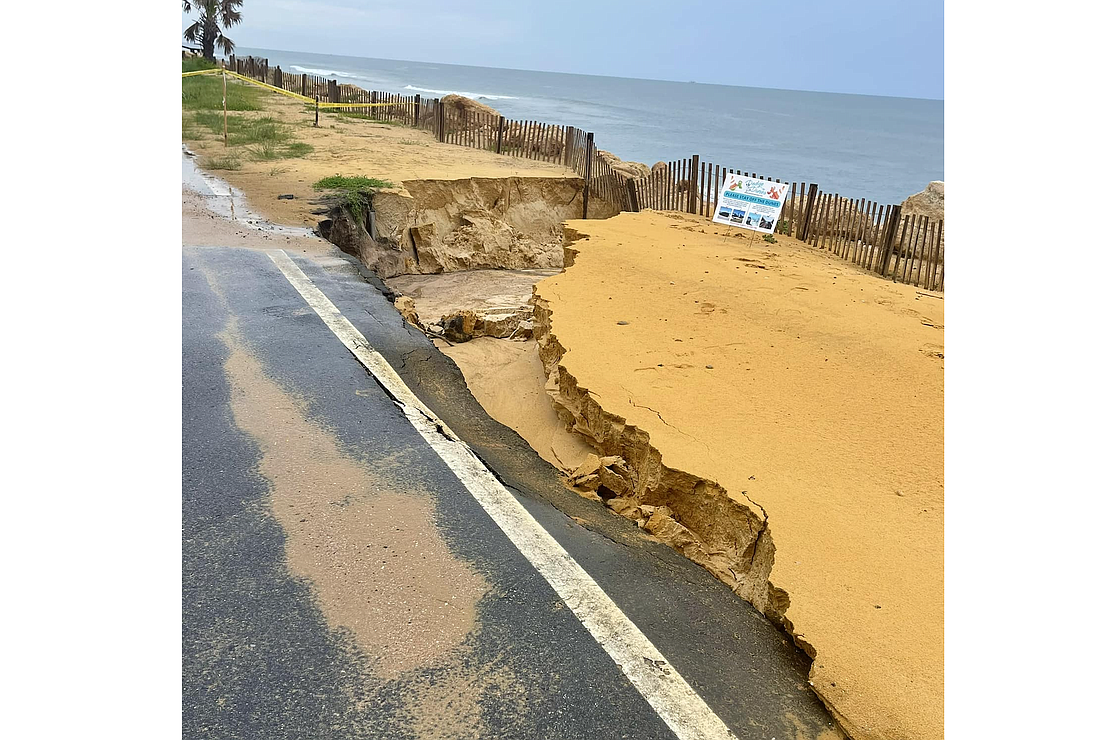This photograph captures a dramatic scene at a beachside area where a road is actively collapsing due to what appears to be severe water erosion. The image prominently features a road that runs parallel to the ocean, which is visible in the distance, stretching to the horizon. This road has large cracks and sections caving in, likely caused by rainwater or flooding that has washed away the underlying sand, creating a pronounced ravine that cuts through the landscape. The sandbank adjacent to the road has been significantly eroded, and the water has created a path leading towards a small, now partially fallen, wooden fence that separates the collapsing area from the rocky shoreline. A warning tape is strung around the perimeter of the affected area, highlighting the danger. A sign—though indistinguishable in text—is also visible, presumably cautioning passersby. The weather appears rainy, adding to the sense of an ongoing natural event. A distant palm tree on the left adds to the coastal ambiance. This image starkly illustrates the destructive force of nature on human infrastructure.